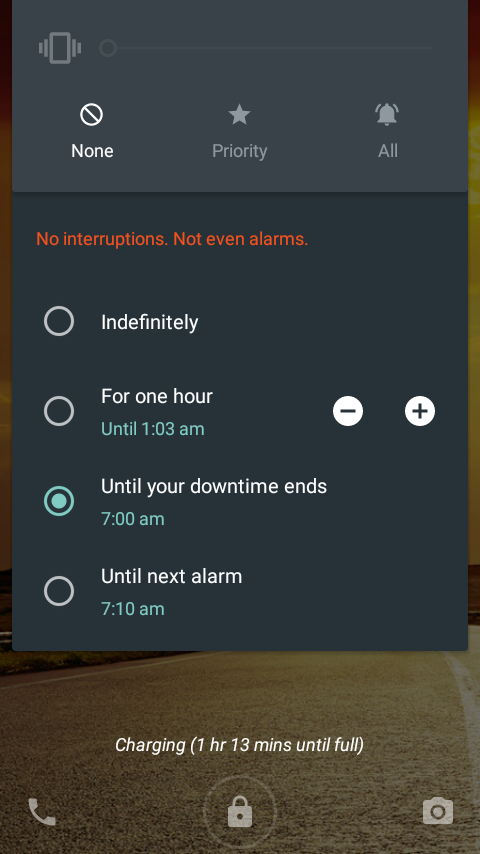Certainly! Here's a more descriptive and detailed caption for the image:

---

The image showcases the "Do Not Disturb" settings on a smartphone screen. The top portion of the screen is shaded in dark gray, featuring a small gray cell phone icon. Below this, a fine line separates the upper section from the options area.

On the left, the word "None" appears in white text, accompanied by a white circle with a diagonal line through it, representing the option to receive no notifications. In the center, the word "Priority" is displayed in gray, beneath a filled-in gray star icon, indicating a setting that allows only priority notifications. On the right, the option "All" is presented in gray text next to a gray bell icon, allowing all notifications.

The background below this section switches to black. At the top of this area, a red text message states, "No interruptions, not even alarms." This is followed by a list of four time-related options:

1. "Indefinitely" – without further details.
2. "For one hour," with a green annotation stating, "Until 1:03 AM."
3. "Until your downtime ends," with an additional green note, "7 AM." This option is selected, as indicated by a filled-in green circle next to it.
4. "Until next alarm," annotated in green with "7:10 AM."

To the right of "For one hour," two white circles with a minus and plus sign allow for adjusting the duration.

Beneath these settings, the background changes to brown. Centrally located, it reads "Charging" with a note in parentheses, "1 hour 13 minutes until full."

At the bottom of the screen, a gray telephone icon is situated on the far left. In the middle, there is a gray lock icon encircled faintly. To the right, a camera icon in gray completes the bottom row.

---